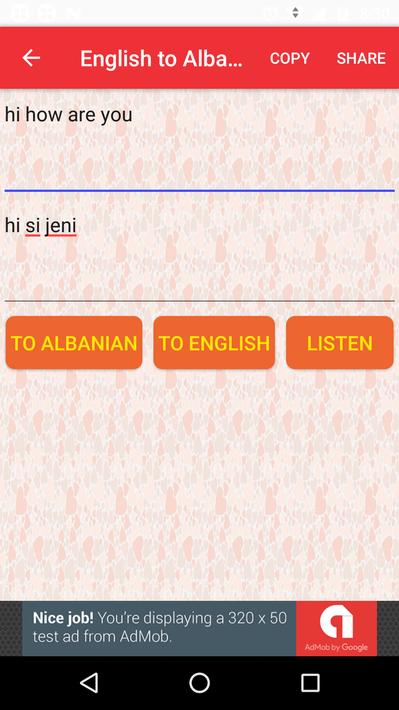This image displays a mobile phone app interface designed for language translation. The background features a patterned peach-colored design. At the top, there is a prominent red header with the title "English to Alba," seemingly indicating translation from English to Albanian. Within this header, text options labeled "Copy" and "Share" are positioned to the right, while a left-pointing arrow is located on the far left.

Beneath the header, the phrase "hi how are you" is shown, presumably the text to be translated. Directly below this text, a bright blue horizontal bar separates the original text from the translated output. The translation appears as "hi see Jenny," likely the Albanian translation of the initial phrase.

Further down, three boxes with an orange background and yellow text display the options "To Albanian," "To English," and "Listen," providing additional translation functionalities. The lower section of the interface contains substantial empty space showcasing the patterned background.

Towards the bottom of the screen, an advertisement declares, "You're displaying a 320 by 50 text or test ad from AdMob." The lowest part of the interface features three icons: a triangle, a circle, and a square, possibly representing navigation or action buttons.